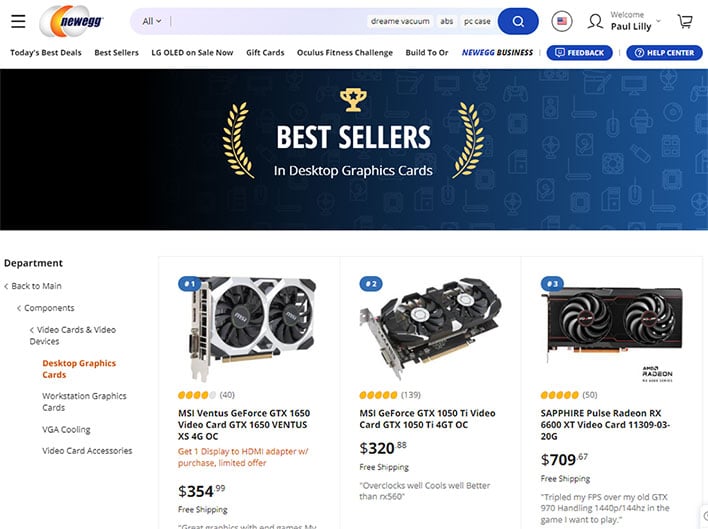This screen capture from the Newegg website showcases its interface and product offerings in great detail. In the top left-hand corner, three black lines indicate a drop-down menu. Adjacent to this is the Newegg logo featuring three interconnected eggs—two white eggs on either side of an orange one, with the word "Newegg" emblazoned above them.

Centered at the top is a search bar with a drop-down menu labeled "All." The search bar contains placeholders like "Dream Vacuum, ABS, PC Case," and a blue magnifying glass icon for initiating searches. On the upper right-hand side, the user's account name, "Paul Lilly," is displayed alongside icons for an account and a shopping cart.

Below, a subheader offers various clickable tabs, including "Today's Best Deals," "Best Sellers," "LG OLED On Sale Now," "Gift Cards," "Oculus Fitness Challenge," "Build 2 Or," and "Newegg Business." Adjacent to these is a feedback button and a Help Center button, both in blue.

The main banner beneath the subheader shows two gold leaves flanking a gold trophy, emblazoned with "Best Sellers" and "Desktop Graphic Cards." Displayed below this banner are three specific graphics cards: the MSI VITNESS GeForce GTX 1650 priced at $354.99, the MSI GeForce GTX 1050 Ti at $320.88, and the Sapphire Pulse Radeon RX 6600 XT listed for $709.67.